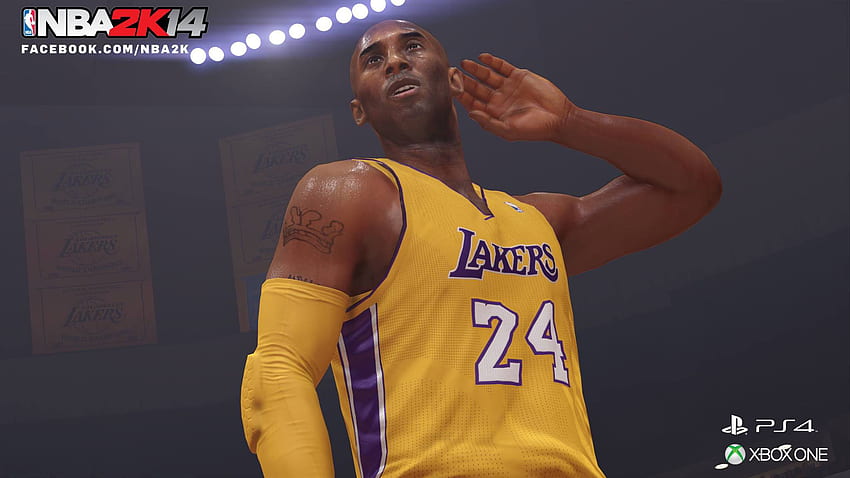The image is a screen capture from the Xbox game NBA 2K14, prominently featuring a simulated depiction of the legendary basketball player Kobe Bryant. Dressed in the iconic yellow Los Angeles Lakers jersey, Bryant's uniform is adorned with "Lakers" written in bold purple letters on the front. His jersey also displays the number 24 in white. He sports a matching yellow sleeve on his right arm. The background of the image is a plain gray, with the NBA logo and the words "NBA 2K14" emblazoned in white, blue, and red text at the upper left corner. Beneath the logo, it reads "facebook.com/NBA2K" in white. Diagonally aligned, several small circles of light are arranged in a row. In the lower right corner, the logos for Xbox PS4 and Xbox One are visible.